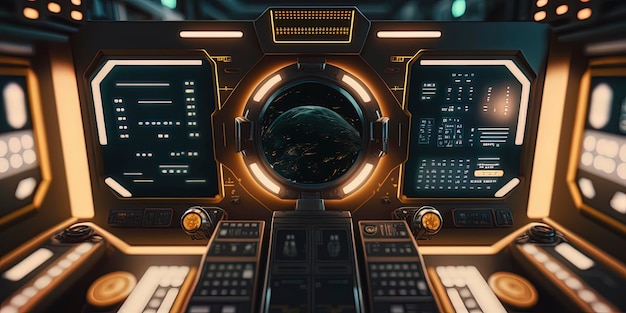The image portrays a digitally created scene of the inside of a spaceship or a rocket. It is a horizontally rectangular, borderless image dominated by the primary colors of blue, white, light tan, and gold. The central focus is a lit-up circular view window through which a planet, possibly Earth, is visible. Surrounding this are an array of brightly lit lights and digital consoles. On either side of the window are two main digital consoles: the left one displaying lines and dashes, and the right one containing additional, albeit unreadable, text. The bottom of the image features a couple of black control consoles. The background includes blurry blue lights, contributing to the futuristic ambiance. The design is cleanly symmetrical, creating a sense of balance and organization within this technologically advanced setting.